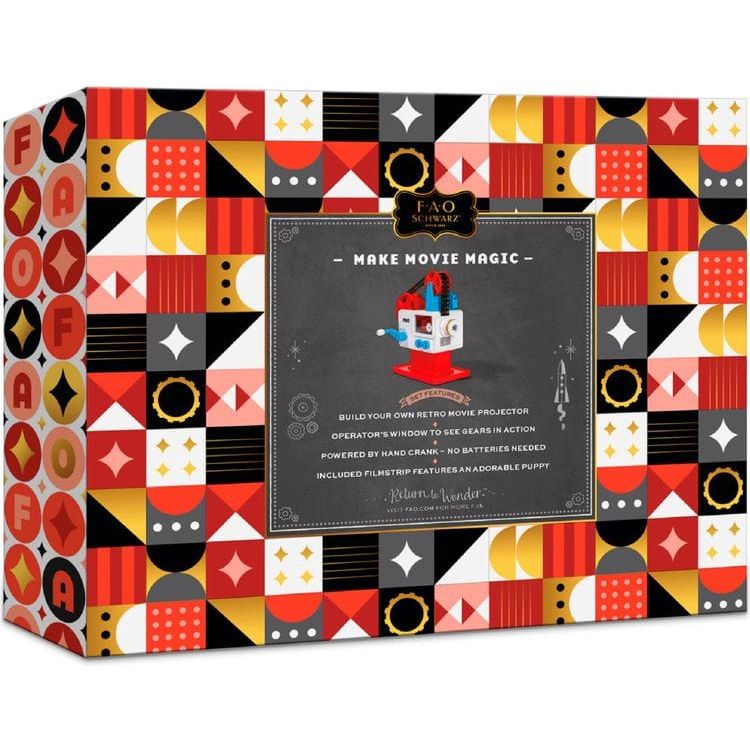This image displays an intricately designed retro-style packaging for a product from FAO Schwartz, prominently labeled on the box. The packaging is characterized by its vibrant and colorful geometric patterns, comprising squares and circles in various colors and designs that repeat to create an eye-catching visual. In the center, a bold, black emblem with gold accents features the FAO Schwartz logo. Directly beneath this emblem, the box has a light black background with a white border and bold white lettering that reads "Make Movie Magic."

The prominent captions and descriptions indicate that the box contains a toy movie projector kit labeled "Build your own retro movie projector. Operator's window to see gears in action. Powered by hand crank. No batteries included. Included filmstrip features an adorable puppy." There's also a charming illustration of a vintage-style hand-crank camera, colored in red, white, and blue. The entire packaging design suggests it can be given as a present without additional gift wrapping, enhancing its appeal as a thoughtful and nostalgic gift item. The product exudes a vintage charm, suggesting it has been around for a few decades, and stands out against the plain white background of the image.